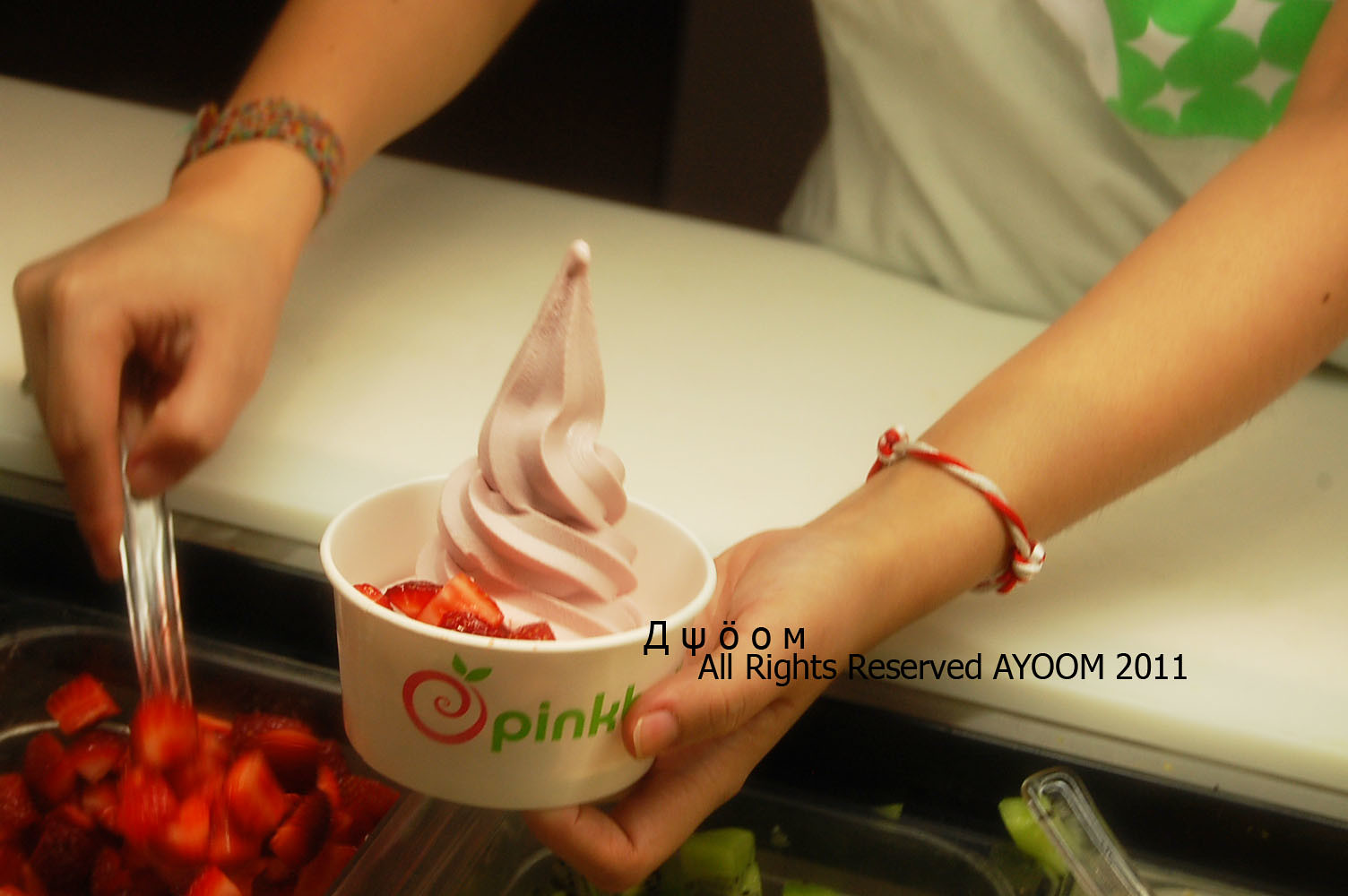The photograph, dated 2011, depicts a close-up view of a young woman, likely a worker or self-serve customer, preparing a dessert at a buffet. She is wearing a white t-shirt with a green design and has both wrists adorned with two bracelets, one thin and red-and-white and the other thicker and multicolored. The image focuses on her hands and torso; her right hand is using a metal spoon to scoop sliced strawberries from a metal container into a small white cup labeled "pink" and featuring the logo "AAUM." Various metal tubs containing other ingredients, such as fruits and vegetables, are visible below the counter. The woman’s left hand holds the white tub, which contains soft-serve ice cream topped with strawberries. A white foam piece is also seen on the counter in front of her. The photograph includes a watermark reading "All Rights Reserved, AAUM, 2011." The woman has a fair, Caucasian complexion.